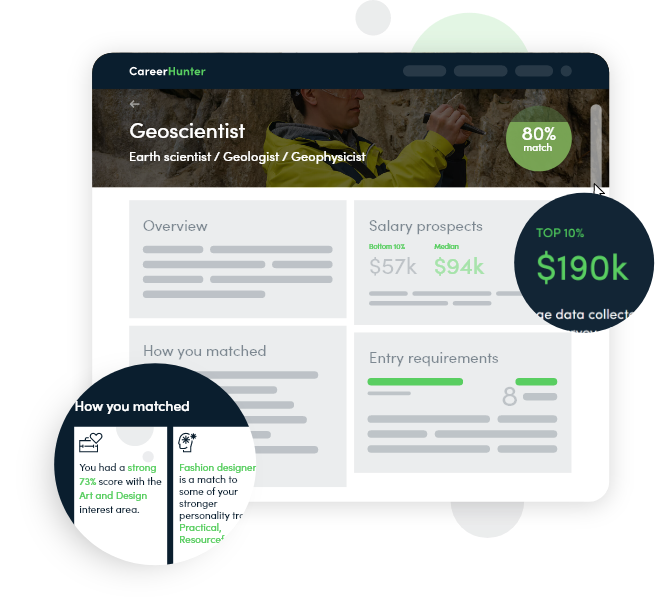This is a detailed screenshot of a CareerHunter webpage. The black top header of the webpage prominently displays the name "CareerHunter," with "Career" in white and "Hunter" in green, forming a single word. Below the header, there is a bold title, "Geoscientist," accompanied by an image of a man dressed in a yellow jacket with a hoodie, painstakingly engraving something onto a stone wall. To the right of this image, a green circle indicates an 80% match for the user.

The main body of the webpage has a clean, white background and features four distinct gray squares, each summarizing different aspects of the Geoscientist career. 

1. The first square (from the left) is titled "Overview."
2. The second square, titled "Salary Prospects," provides detailed salary data. It highlights that the bottom 10% earn $57,000, the median salary is $94,000, and the top 10% make $190,000. These figures are set within a solid dark green circle with light green text.
3. The third square is labeled "How You Matched," showing how well the user’s profile aligns with the career.
4. The final square is titled "Entry Requirements," which likely outlines what qualifications are needed to pursue this career.

Additionally, the detailed match section features a zoomed-in portion that expands on the specific user’s alignment with the Geoscientist role.